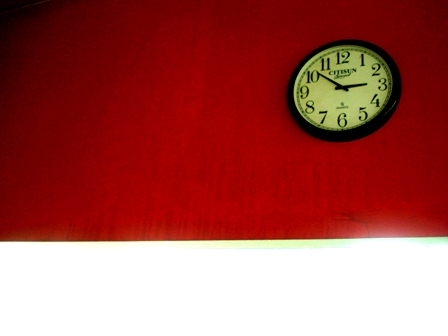In this image, a striking red wall serves as the backdrop for a classic, black-framed clock. The clock features a white face, which prominently displays black Arabic numerals from 1 to 12, arranged in their usual positions around the dial. At the center of the clock face, two sleek black hands indicate the hours and minutes, while the clock notably lacks a seconds hand. Above the hands, faint black text is visible, but it is too small to decipher. Similarly, there is additional black text beneath the hands, which is also too small to read. The simplicity and contrast of the clock against the bold red wall make for a visually captivating image.